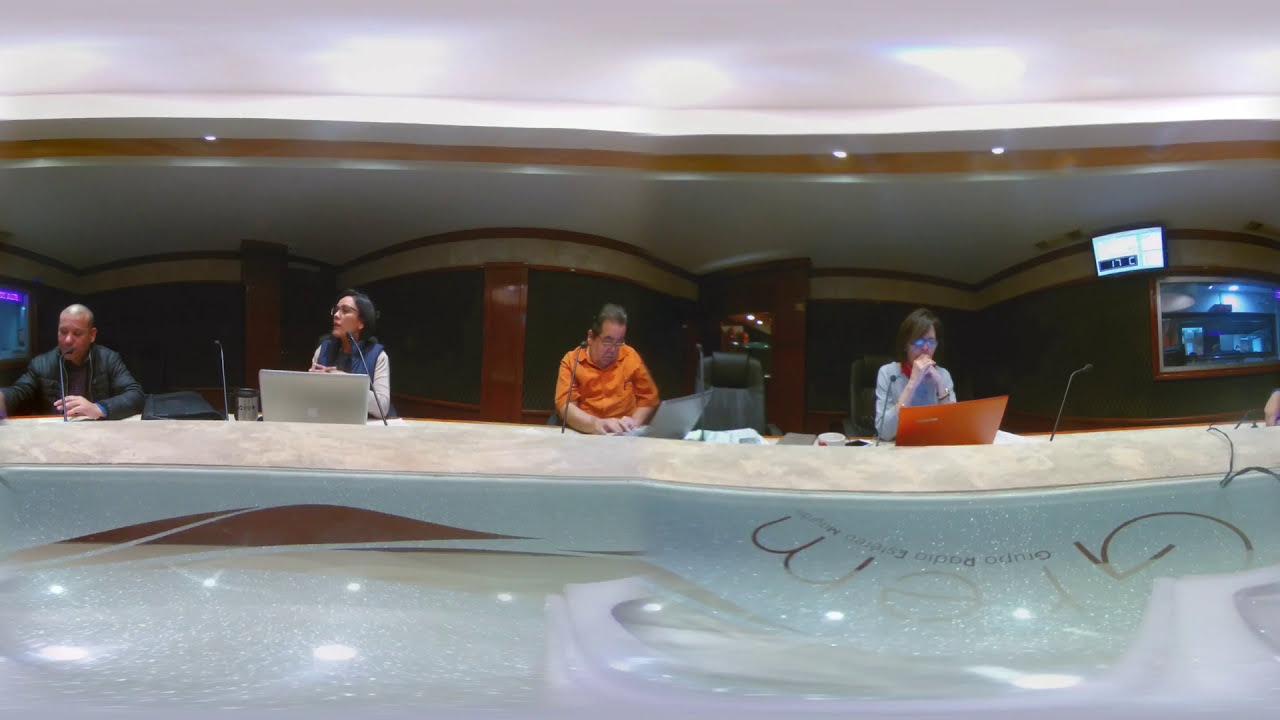In this color photograph, four individuals are seated at a marble countertop equipped with laptops and microphones, participating in what appears to be a business conference or presentation. The setting is a modern room with a white ceiling, featuring architectural wall projections and possibly overlooking a venue, suggested by the box seat-like ambiance.

The man on the far left, around 45 years old, is wearing a black long-sleeve shirt and is engaged in speaking into a microphone. Centrally towards the left is a woman in a blue vest and white long-sleeve shirt, looking up to her left, and working on a silver laptop. Next to her sits another man, approximately 50 years old, in an orange shirt. He has dark hair, glasses, and is focused on his laptop. Toward the right at the counter, a woman around 35 years old in a light blue shirt has her hands clasped in front of her face and is peering down at her laptop. Both women are wearing glasses.

In the background, a monitor is mounted on the wall, with a white image displaying the letters "G-R-E-M" in a curved arrangement followed by some text in a foreign language. The photograph is taken in landscape orientation with a panoramic view, capturing the detailed and focused ambiance of the scene.